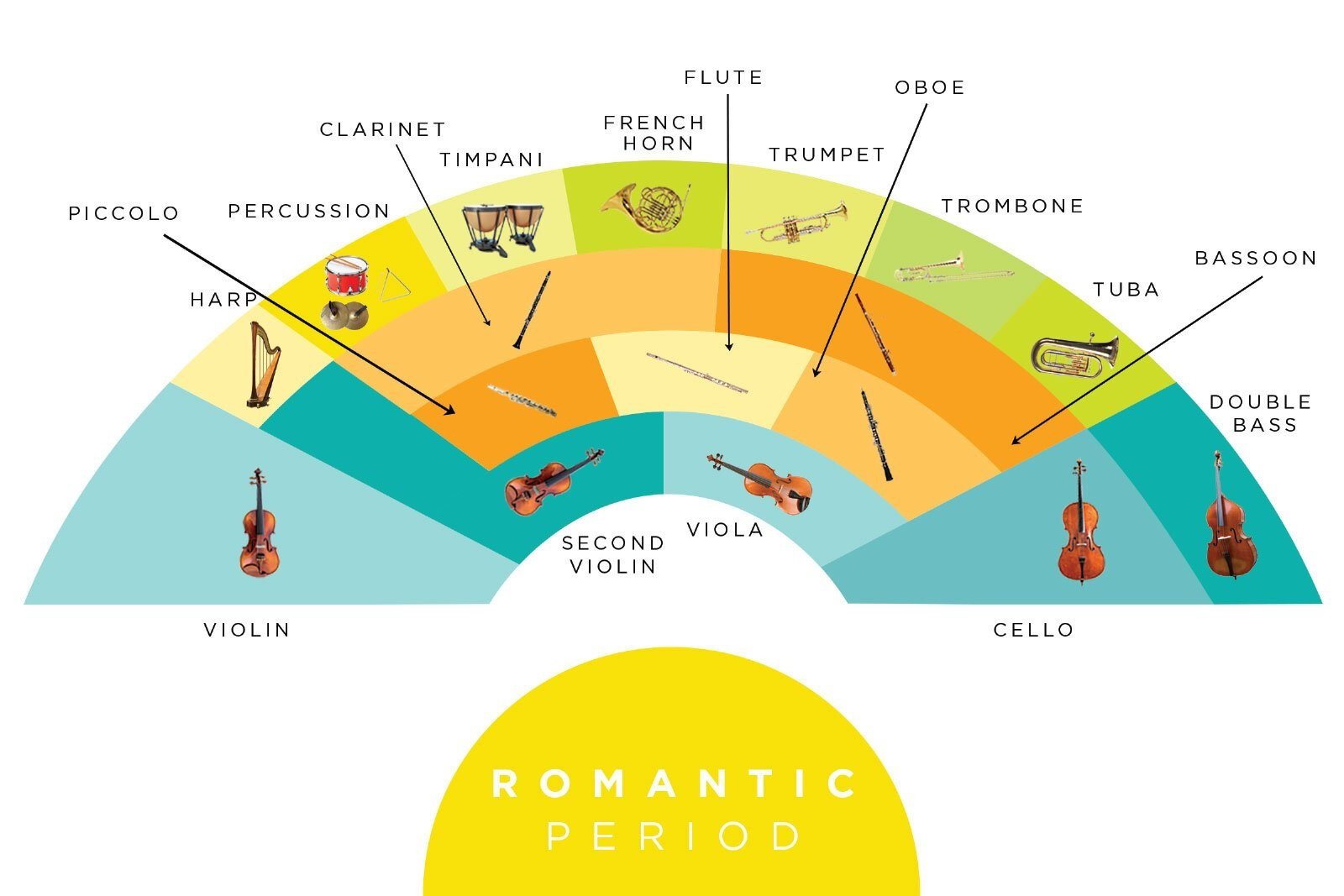The image depicts a detailed and colorful orchestral seating chart, prominently displaying a yellow semicircle at the bottom with white text that reads "Romantic Period." Above this, a multicolored semicircle chart illustrates the seating arrangement of various instruments, ranging from light blue to dark blue, light green, orange, dark orange, and yellow. Each section contains labeled images of instruments accompanied by black text, with some names pointing to their corresponding images via arrows.

From left to right in the front row, labeled as the second violin and viola section, the semicircle's design spans out to depict instruments in successive rows. In the second row from the front, there are the piccolo, flute, and oboe. The next row up features the clarinet and additional oboes. In the back rows, the chart positions the larger and lower-pitched instruments: the harp, percussion, timpani drums, French horn, trumpet, trombone, tuba, double bass, and cello. The layout systematically represents the arrangement within an orchestra during the Romantic Period, showcasing where each musician would typically be seated in a concert setting. The entire image is set against a white background.